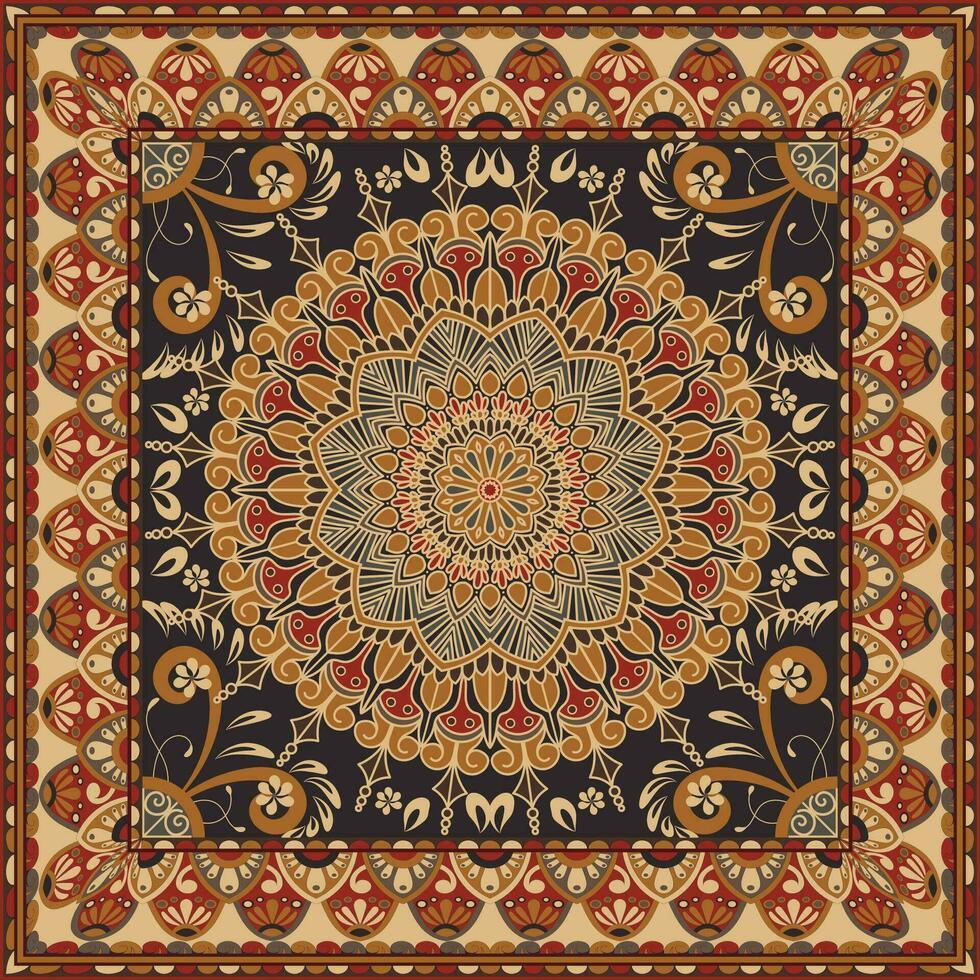The image depicts a square-shaped, Persian or Middle Eastern-style tapestry with rich detailing and vibrant colors. The primary colors used are burnt sienna, charcoal black, burgundy, white, and accents of pale olive green. At the center lies a prominent mandala-style design, composed of intricate layers of shapes and colors radiating outward. This central motif emerges from a black background and is framed by decorative borders featuring patterns resembling half Easter eggs adorned with varied designs. The outermost edge of the tapestry consists of semi-circles in colors that echo the inner tapestry's palette.

Intricate shapes, including circles and ovals, grow larger as they move toward the edges of the rug, with an inner square framing these circular motifs. Notably, the center of the mandala features a face with two red dots and a headdress, surrounded by a line forming another concentric circle. The design includes floral elements created from circles, adding to the tapestry's ornate and traditional aesthetic. The colors, while not muted, harmonize well with each other, contributing to the tapestry's cohesive and visually striking appearance.